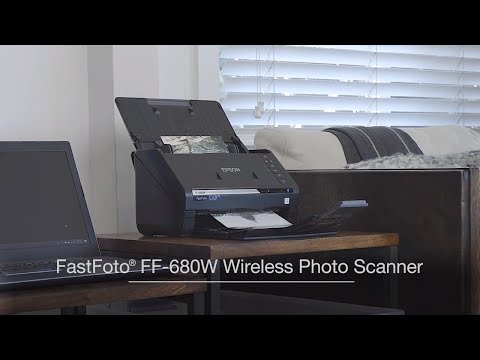This product image showcases the Epson Fast Photo FF-680W Wireless Photo Scanner placed on a small wooden table with metal legs. The black scanner, with an Epson logo around the center and the product name labeled in white sans serif font at the bottom, is actively scanning an item, with the paper visibly emerging from the other end. To the left of the scanner, a black laptop partially appears on a shorter table. The setting features a black and white leather couch with a fluffy rug, positioned next to the wooden table. Behind the couch, a large window with closed blinds allows daylight to filter through, casting a soft light on the white walls of the room. The image has black bars at the top and bottom, suggesting it may be a video screenshot.